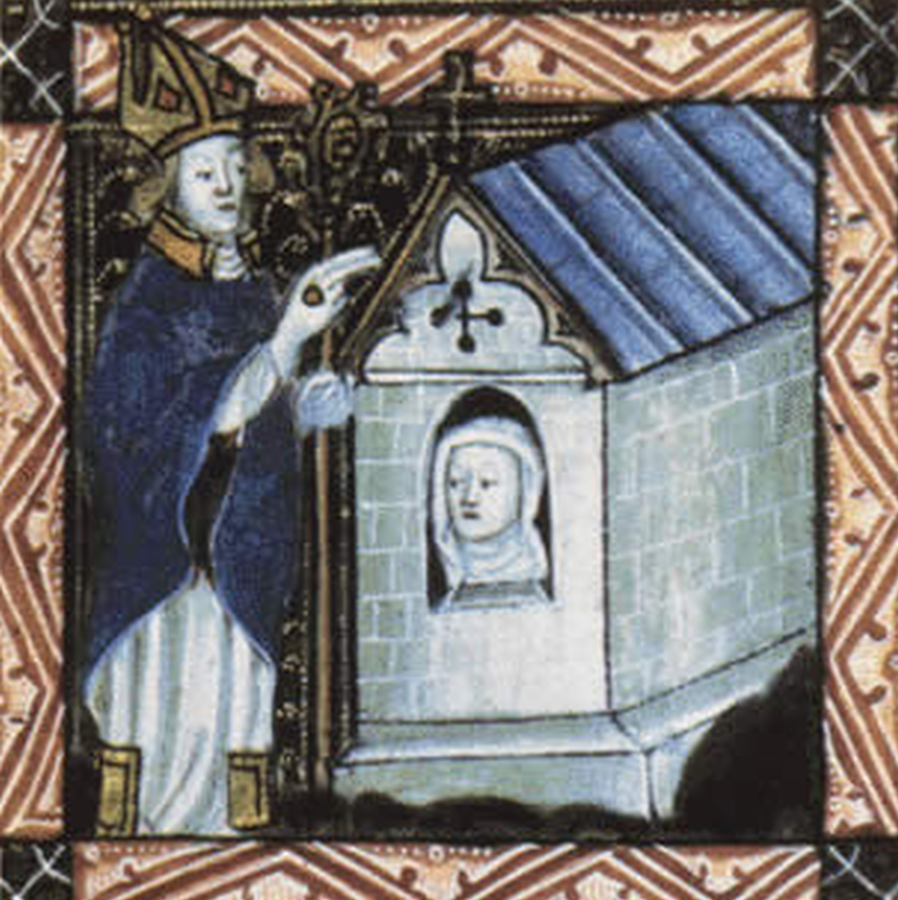The image appears to be an old, detailed painting with a religious theme, framed by a pattern of peach and rust-red zigzag lines. Dominating the left side of the painting is a figure resembling a priest or possibly a pope. He wears an elaborate gold hat adorned with red emblems, a blue garment draped over a white robe, and a ring on his outstretched hand. In his other hand, he holds a staff, suggesting his high rank within the church. The background features a complex brown pattern with zigzag lines interspersed with black. To the right of the priest stands a small, brick building with a blue roof and a cross on top. A window in the building reveals the upper part of a woman dressed in white. The scene appears reminiscent of a stained glass window from a church, depicting a confessional moment or a significant religious interaction. The overall setting reinforces the sacred and ceremonial atmosphere of the painting.